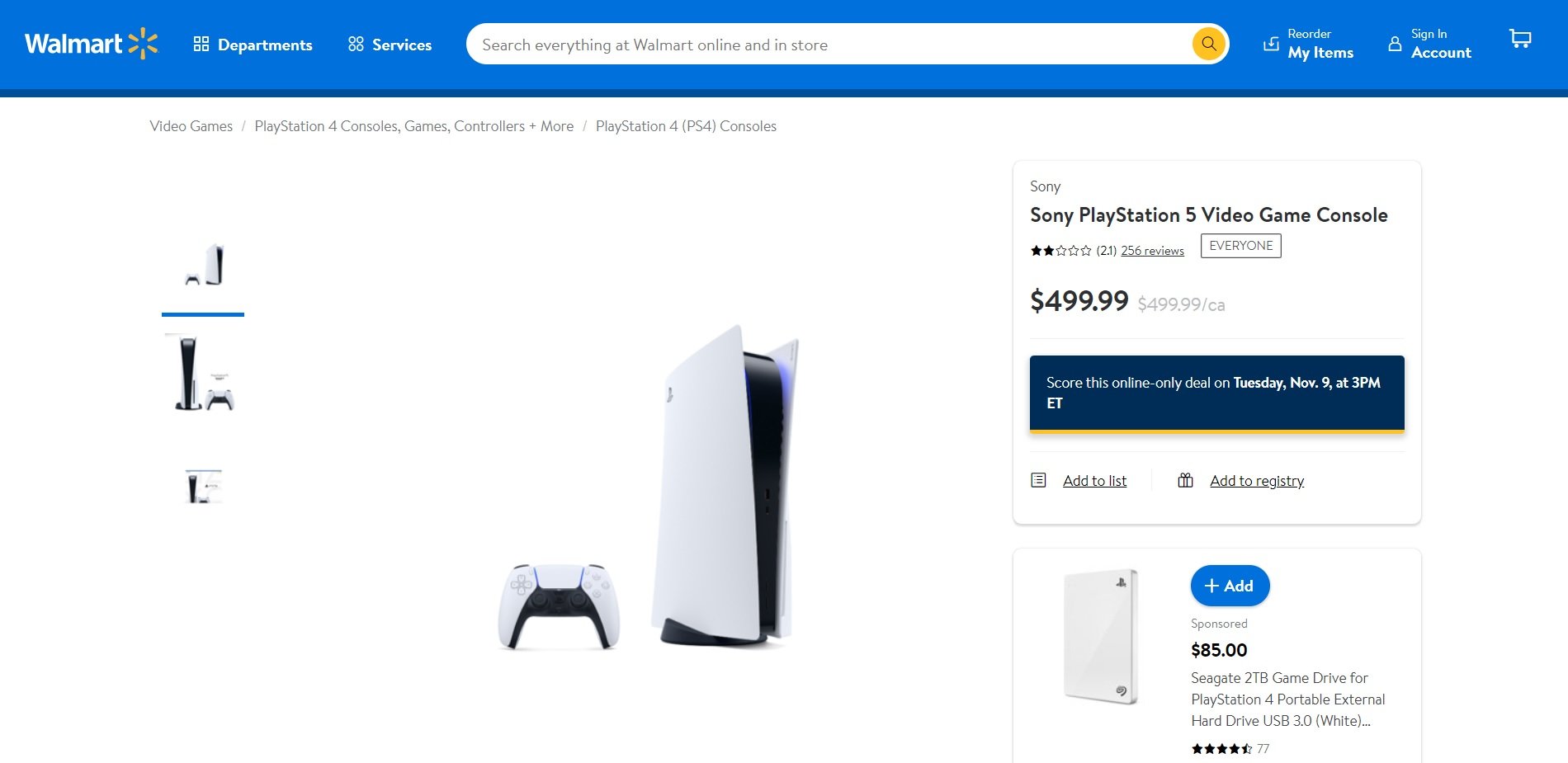This is a screenshot of the Walmart website. At the top of the page, the header displays the Walmart logo prominently. Below the header, there are navigation options including 'Departments' and 'Services.' A search bar is positioned at the center of the page with the placeholder text, "Search everything on Walmart online and in-store," accompanied by a magnifying glass icon. 

On the right side, there are options labeled 'My Items' and 'Sign In Account.'

The main content features a section dedicated to video games, focusing on PlayStation products. This includes image displays, prices, and ratings for various items. One prominent product listed is the 'Sony PlayStation 5 Video Game Console,' priced at $499.99. Below this product, there are options to 'Add to List' and 'Add to Registry,' as well as a note indicating the item is ad-sponsored.

Also featured is the 'CA-21B Gem Drive for PlayStation 4,' described as a portable external hard drive with USB 3.0 in white, priced at $85.00. This product has a five-star rating based on 77 reviews.

Similarly, the Sony PlayStation 5 console has a five-star rating from 211 reviews, emphasizing its popularity and customer satisfaction.